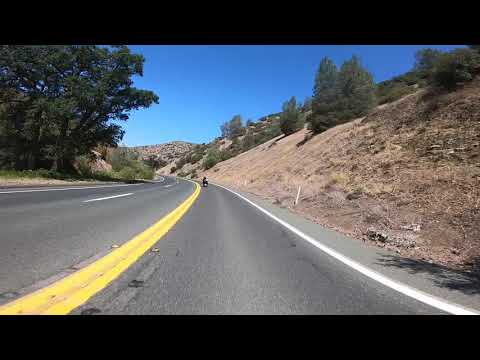The photograph captures an open stretch of a lonely road under a brilliant blue sky that fades into a lighter hue at the horizon. The road consists of a single lane heading in the right direction and two lanes on the left, divided by solid yellow lines. The right lane is edged by a solid white line, beyond which a motorcycle can be seen in the distance, approaching a curve in what appears to be the bike lane. The road is accompanied by a hilly embankment on the right side, characterized by sandy beige dirt and patches of pine trees and small, green-leaved bushes. On the left side of the road, there's a flat area with more trees closer to the highway and a backdrop of scrub and dirt. There is also a prominent large tree with smaller bushes in front of it, bordering an area that appears to be sand or dead grass. The overall scene is framed within a small rectangular picture with a solid, thick black border.